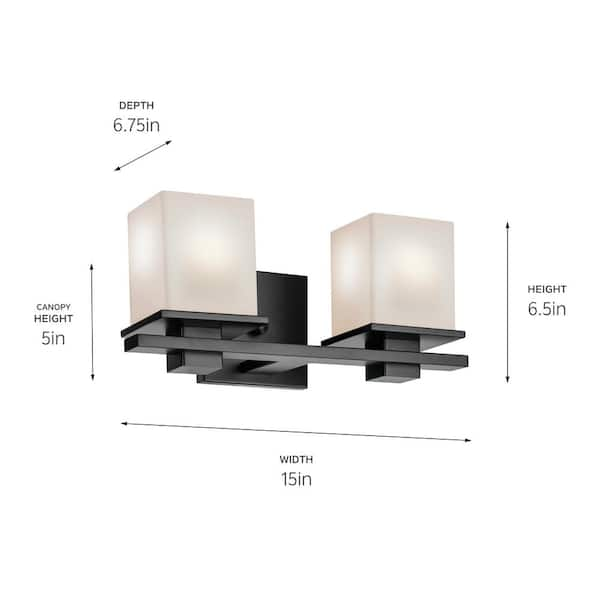This image is a detailed product shot of a black metal hanging wall lamp with two distinct white cube-like lampshades. Each lampshade is positioned on either side of a horizontal black metal bar, which creates a T-shaped structure when viewed from the side. The lamp features prominently labeled dimensions: a depth of 6.75 inches at the top, a canopy height of 5 inches on the left side, an overall height of 6.5 inches on the right side, and a width of 15 inches at the bottom. The canopy height refers to the metal base plate that attaches the fixture to the wall. The image, set against a plain white background, resembles a product picture typical for online listings, such as those found on Amazon. It includes black arrows and text indicating various measurements, enhancing its utility for potential buyers looking for precise spatial requirements.